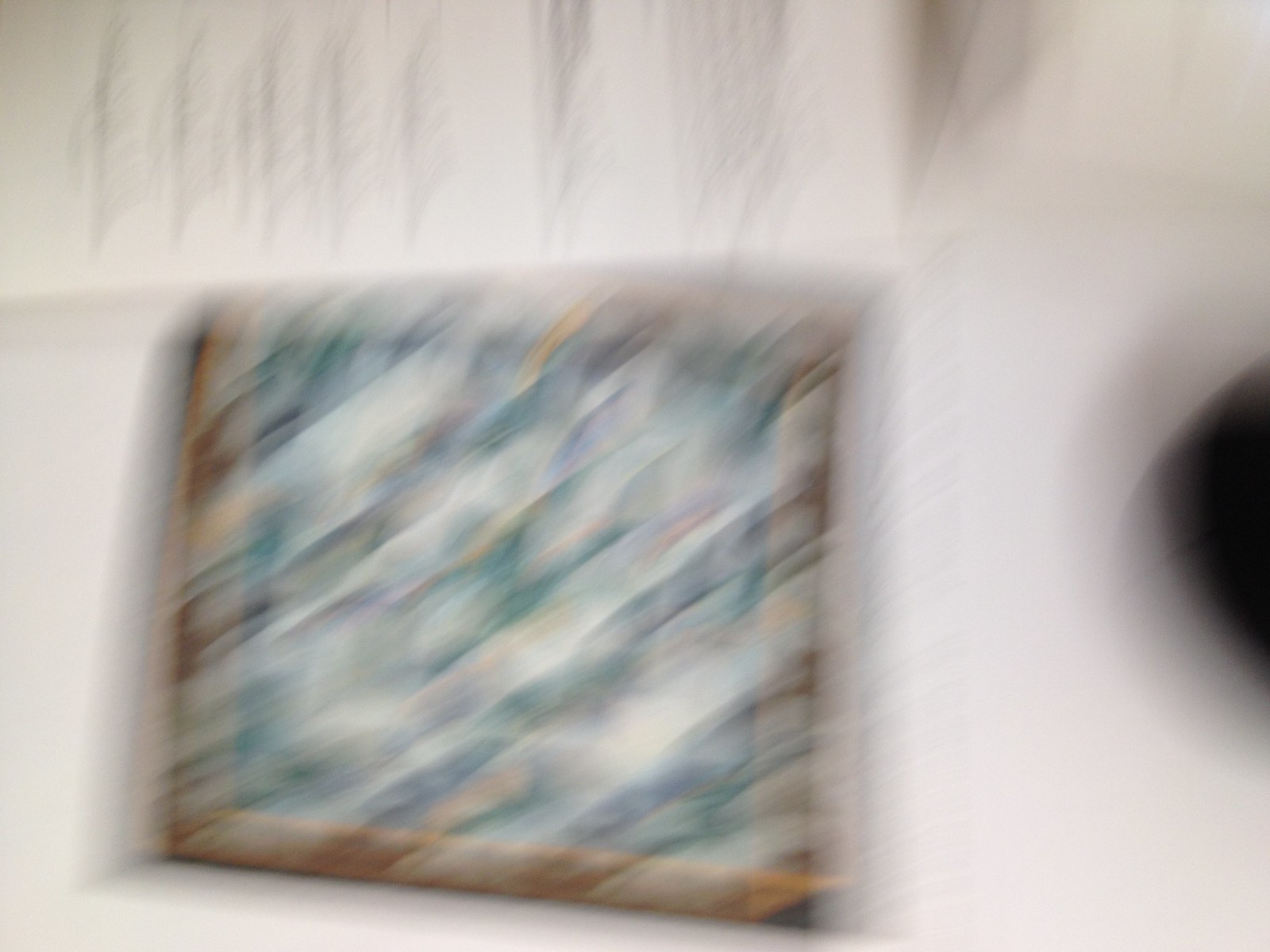The image is very blurry, making it difficult to discern specific details. Dominated by a white background, possibly a wall, there are subtle black accents that create a noticeable contrast. A distinct dividing line suggests a separation between the white wall and a similarly white surface, perhaps a sofa. Centrally located within the image, there seems to be a square object, likely a painting, picture frame, or a carpet with visible colors that include yellow, green, blue, and brown. To the right side of the image, there is a black, half-circle shape that could be an object or part of the decor. The combined elements create an abstract and indistinct composition.